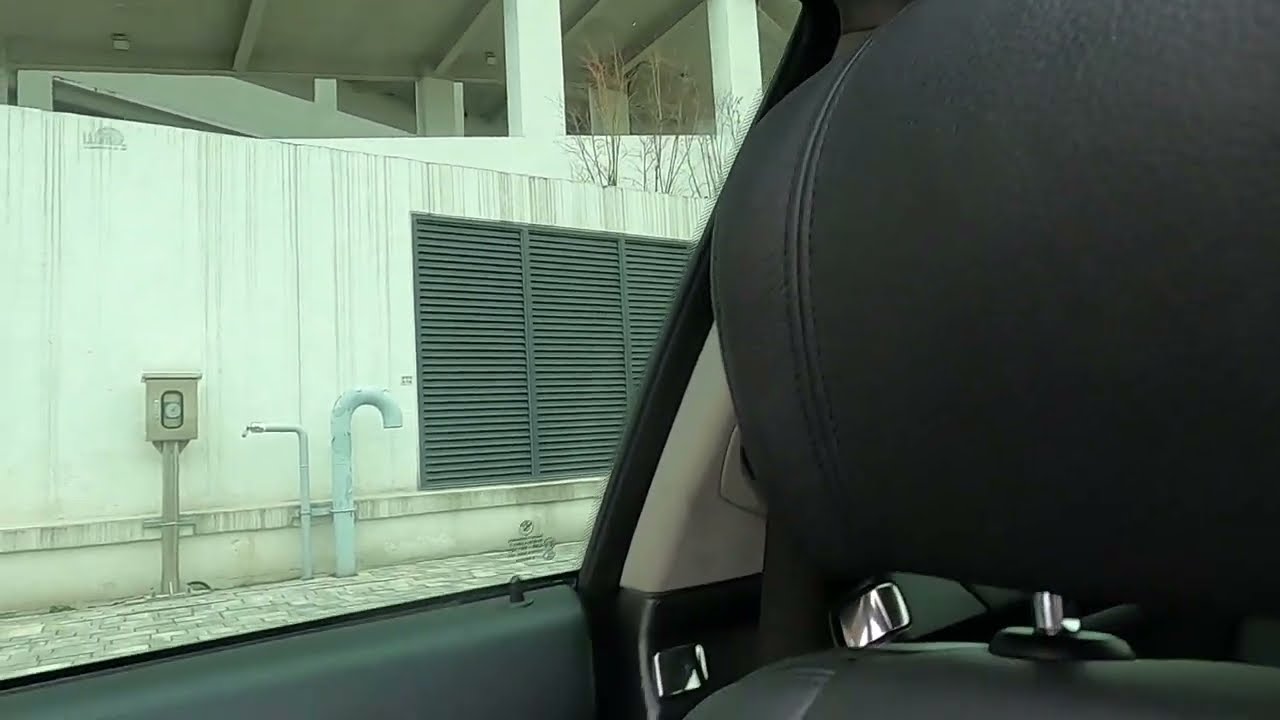This image captures the inside of a vehicle, specifically from the back seat. Dominating the right side of the frame is the black leather headrest of the front seat, while visible details include the car door with its black trim, an unlocked door lock, and the window. Through the window, one can see a cobblestone sidewalk on the left, leading up to a white building exterior. The building features white walls, pillars supporting a second level, a gray meter, and a white pipe or vent extending from the ground. Additionally, some trees are visible in the background, adding a touch of nature to the urban scene. The colors present in the image include off-white, light brown, tan, light blue, black, gray, silver, and touches of purple.